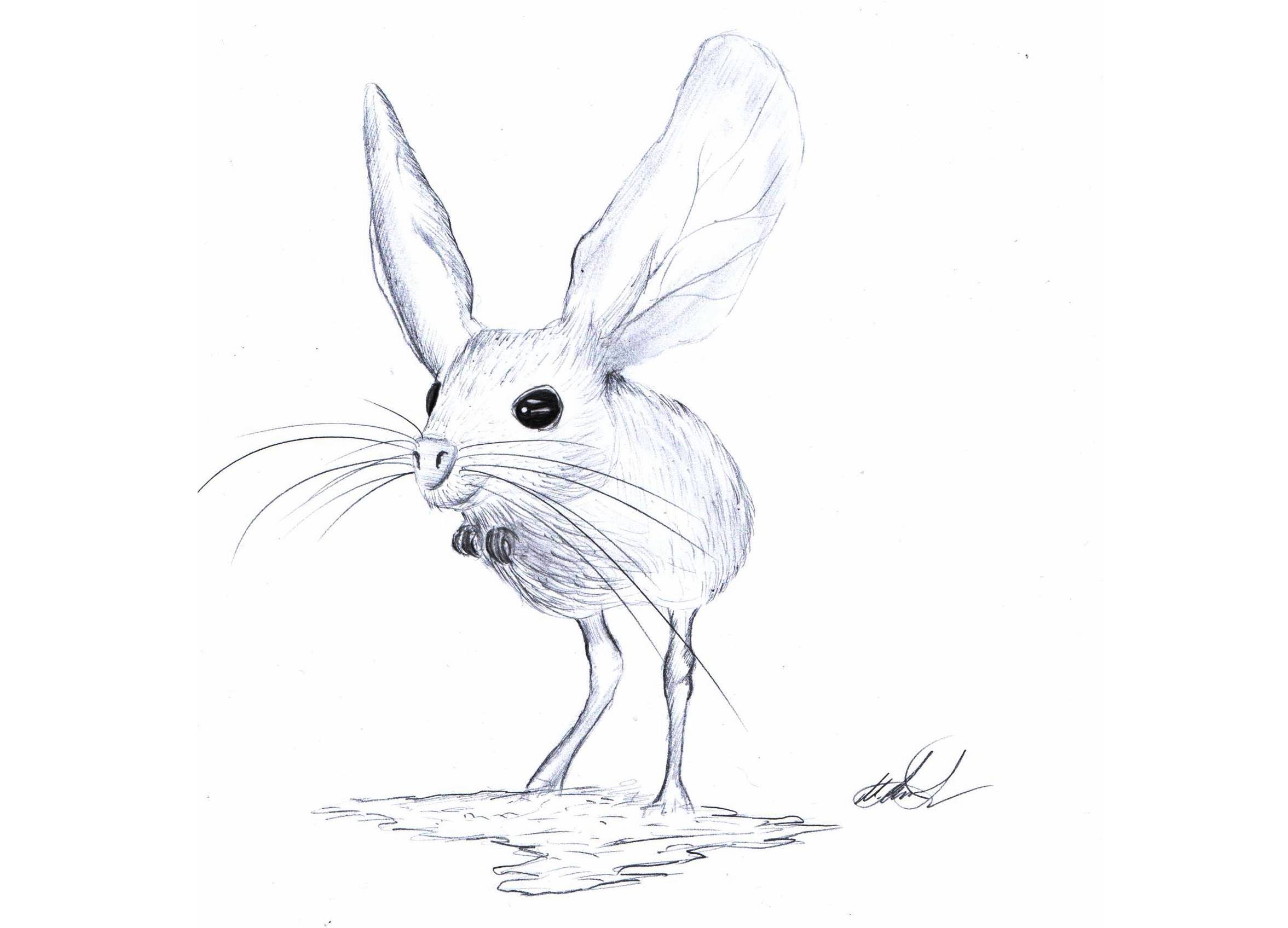This is a hand-drawn pencil illustration of a unique, furry desert mouse-like creature. Standing upright on two long legs—suggestive of those of a rabbit or even a chicken—it appears poised to be a fast runner or high jumper. Its hilariously large, veiny ears, about the size of its entire body, stand tall and pointed upward. The creature's face features dark, black round eyes and exceptionally long whiskers, enhancing its adorableness. It holds its tiny paws curled inward near its chest, reminiscent of a velociraptor. The mouse stands on a small, grassy patch and looks off happily into the distance. The drawing is signed by the artist in the lower right corner, although the signature is illegible. The entire illustration is in black and white, emphasizing the creature's distinct features.